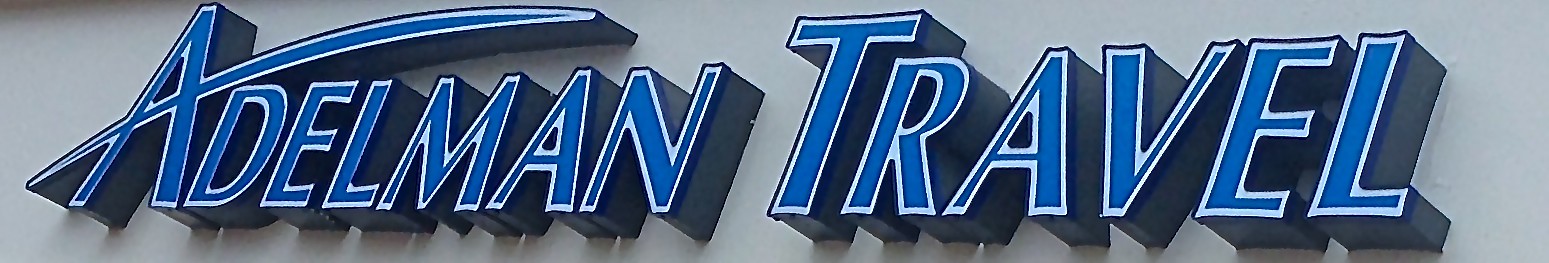The image features a horizontally rectangular sign displaying "Adelman Travel." The text is composed of three-dimensional blue letters with white linings. The underside and outer edges of the letters are dark gray. A distinct curved line originates from the left-hand side of the letter "A" and extends just before the "N" in "Adelman," running along the top of the word. The entire sign is set against a light gray background.